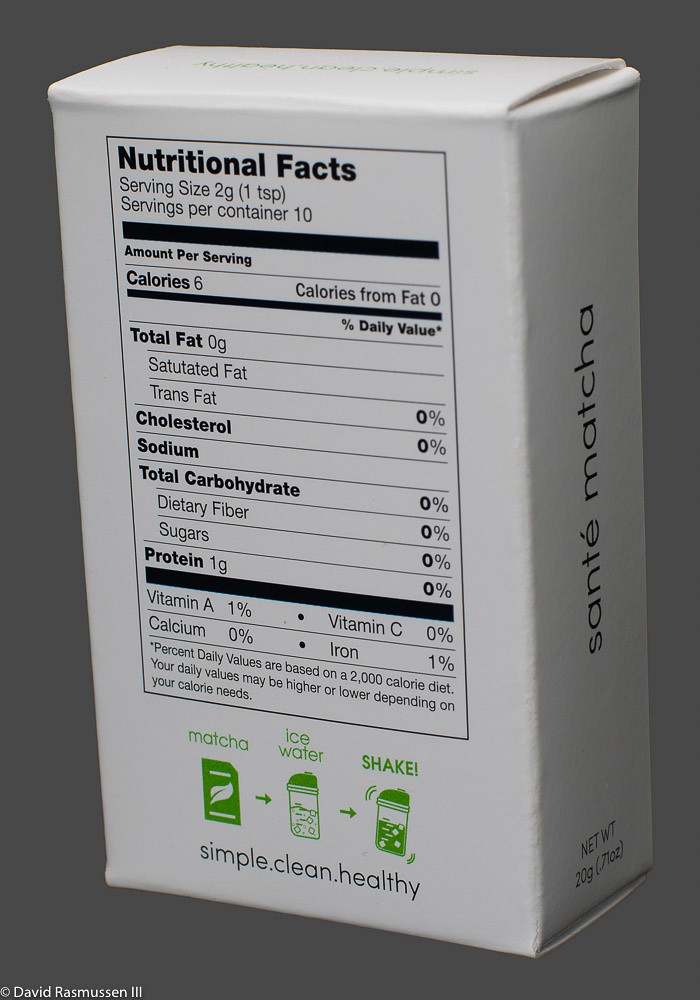This close-up photograph captures the backside of a tea box, presented from an oblique angle that reveals both the back and side panels. The box itself is predominantly white. The side of the box features the text "Sencha Matcha" in black letters. The back panel showcases the nutritional facts label, which indicates that the tea has 6 calories, 1 gram of protein, and zero values for the remaining nutritional metrics. At the bottom of this panel, the slogan "Simple. Clean. Healthy." is prominently displayed. Below the slogan, a straightforward diagram illustrates the preparation method, showing "Matcha" with an arrow pointing to "Ice Water" and another arrow leading to "Shake!" The setting is a neutral gray background, and nestled in the far left corner in tiny white letters is the name "David Rasmussen III."